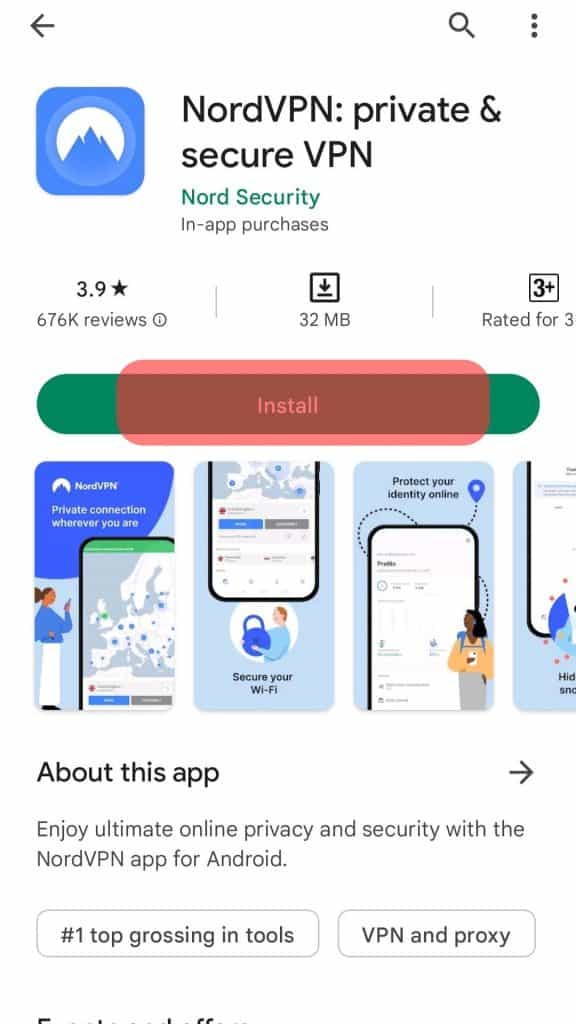This image appears to be a screenshot from a mobile device showcasing the interface of a Google App Store or a similar app marketplace. The screenshot is portrait-oriented and features an interface primarily set against a green and white backdrop.

At the top left, there is a black, left-pointing arrow that functions as a back button. On the top right, there is a magnifying glass icon for search functionality and a vertically-stacked three-dot menu for additional options. Below these icons, the search bar displays the result: "NordVPN, private and secure VPN," accompanied by a thumbnail of the app's icon. 

The NordVPN icon is a blue square with rounded edges. Within the icon, there is a white circle featuring a blue mountain-like structure at its base. Beneath this title, the developer name "Nord Security" is written in green, followed by an indication that the app offers in-app purchases.

Further down, information about the app's rating and details are provided. The app has an average rating of 3.9 stars based on 676,000 reviews, occupies 32 megabytes of storage space, and is rated appropriate for users aged 3 and older. 

Directly below this information is a prominent, green 'Install' button, which is long, oval-shaped, and features white text. This button is partially highlighted by a red, transparent oval shape, suggesting that it is the focal point of interest. Below this area, there is a graphic representation of the phone showing what the app does, which is followed by the text "About This App" in black font, indicating the section for app description and details.

The screenshot seems to be informative and comprehensive, providing potential users with essential details to help them decide whether or not to download the app.